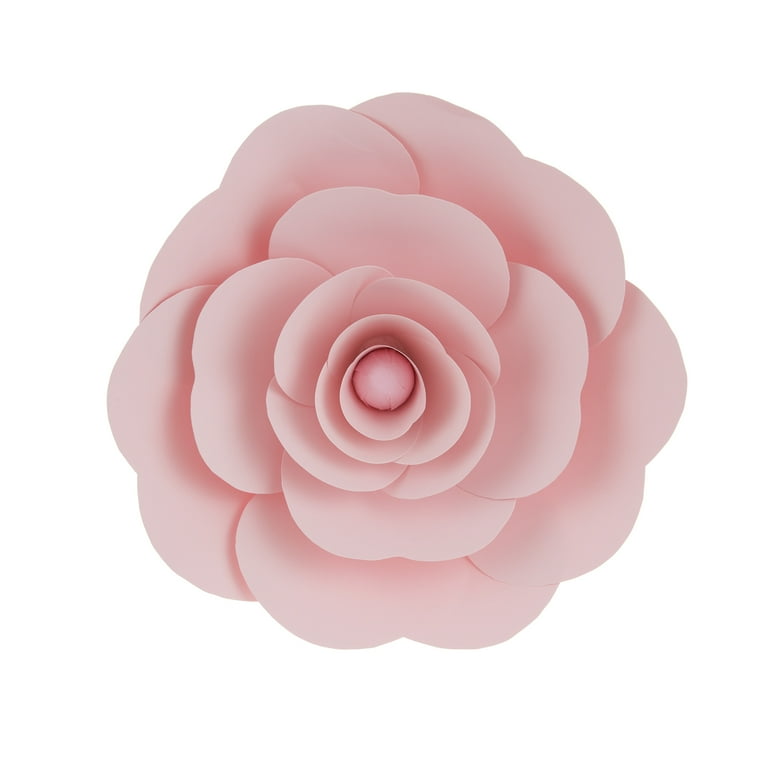The image showcases a close-up view of a blooming pink flower, prominently displayed against an infinite white background. The flower, resembling a rose, peony, or camellia, is centered and takes up the majority of the image space. The petals, lush, full, and healthy, exhibit a gradient in size, with the outer ones being larger. The center of the flower remains tightly bunched, giving way to a rounded, cup-like formation. Each layer of petals casts subtle shadows, enhancing the flower's delicate texture and depth. No stem or leaves are visible, emphasizing the intricate, concentric arrangement of the petals.